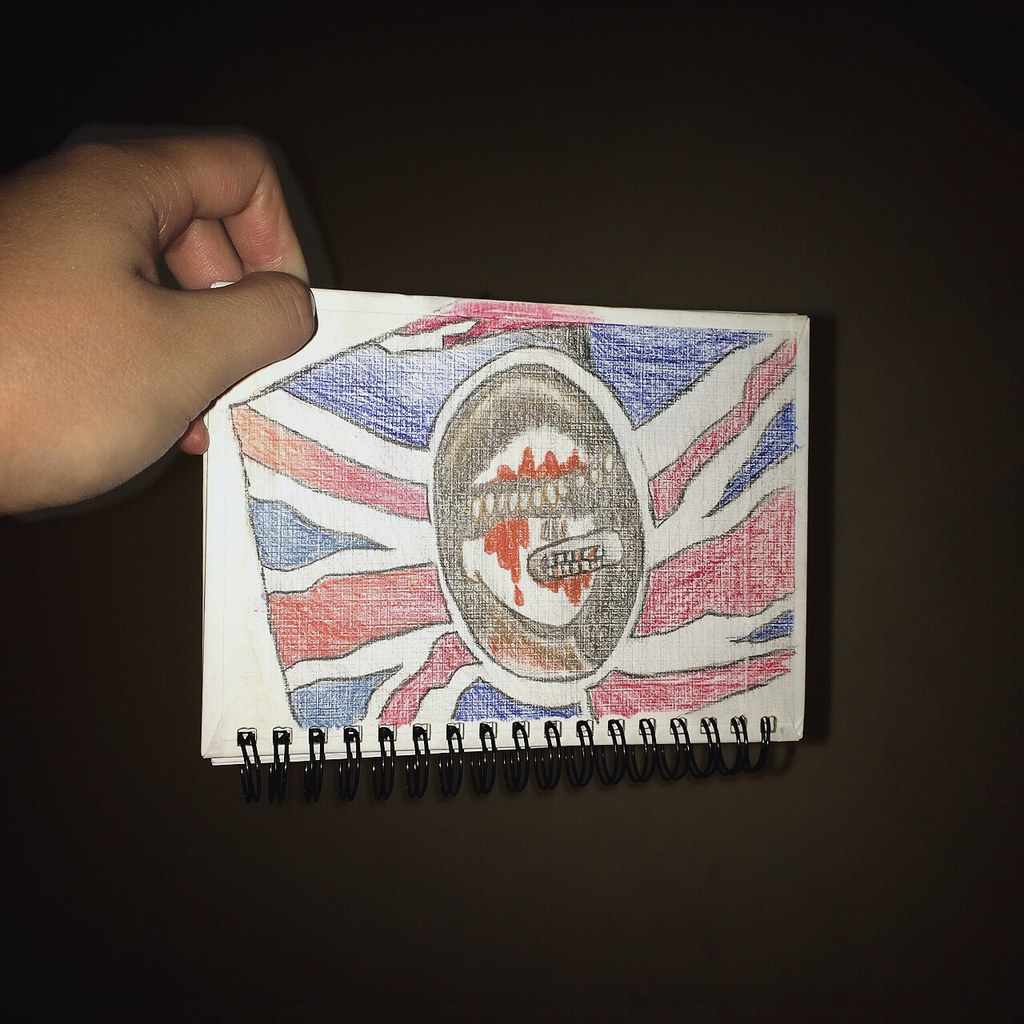In this image, a person's hand is holding up a small sketchpad by pinching the top left corner. The sketchpad features a detailed drawing of the British flag, prominently displayed in the center of the pad. The flag's classic design consists of red and blue fields with white stripes radiating from the center. 

Within the center of the flag, there’s an intriguing circular design resembling a mouth. This circle is black and shaded to appear shiny. Inside the black circle, there's an opening filled with small white circles, further emphasizing the mouth-like appearance. Red markings are also present within the circle, adding complexity to the design.

At the bottom edge of the sketchpad, black rings are visible, binding the pad together. The intricacy of the flag's depiction, combined with the unique central design, showcases the artist's attention to detail.